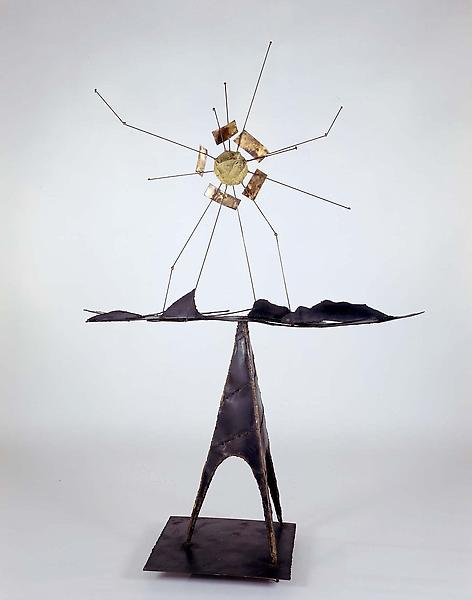The image features a peculiar and intricate abstract sculpture positioned against a grey background, likely within a museum. The sculpture stands on a copper base that supports a triangular, almost Eiffel Tower-like structure, which extends vertically. This structure culminates in a platform that appears to branch out and support a complex, spider-like fixture with approximately nine to eleven spindly legs, radiating outward. Central to the sculpture is a golden medallion or dish adorned with small rectangular pieces that are golden or white with highlights. The sculpture's spiky and multi-layered design combines modern art aesthetics with a blend of metal tones ranging from grey to brown and touches of yellow, resulting in a visually striking centerpiece.